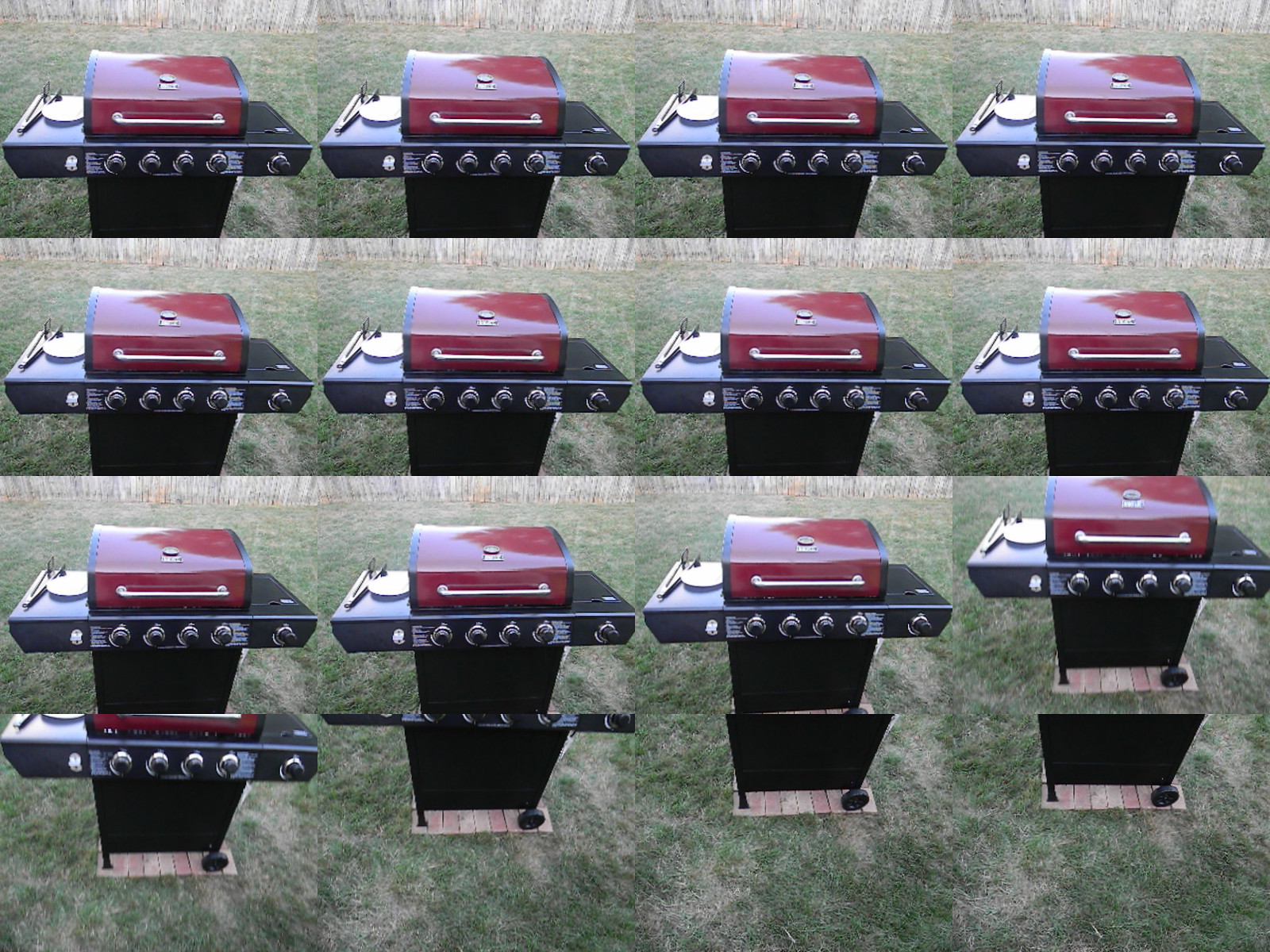The image showcases a grid of 16 barbecue grill photographs arranged in four rows and four columns, taken from slightly different angles. The focal subject is a four-burner grill with a distinctive rich woody red lid adorned with a silver handle and a built-in temperature gauge on top. The grill features a black rectangular base and a side burner on the right. There are five control knobs located on a black strip just below the main cooking surface. The left shelf holds a pair of silver tongs with black rubber tips and a small white saucer. The grill appears to be placed on wooden boards laid over a grassy area, which is worn down from substantial foot traffic. The background in all photos is a blend of green grass with patches of light-colored dirt. The arrangement of the images highlights different parts of the grill, with the bottom row of photographs primarily displaying the grill's lower black base, including a wheel on the right and a leg on the left.